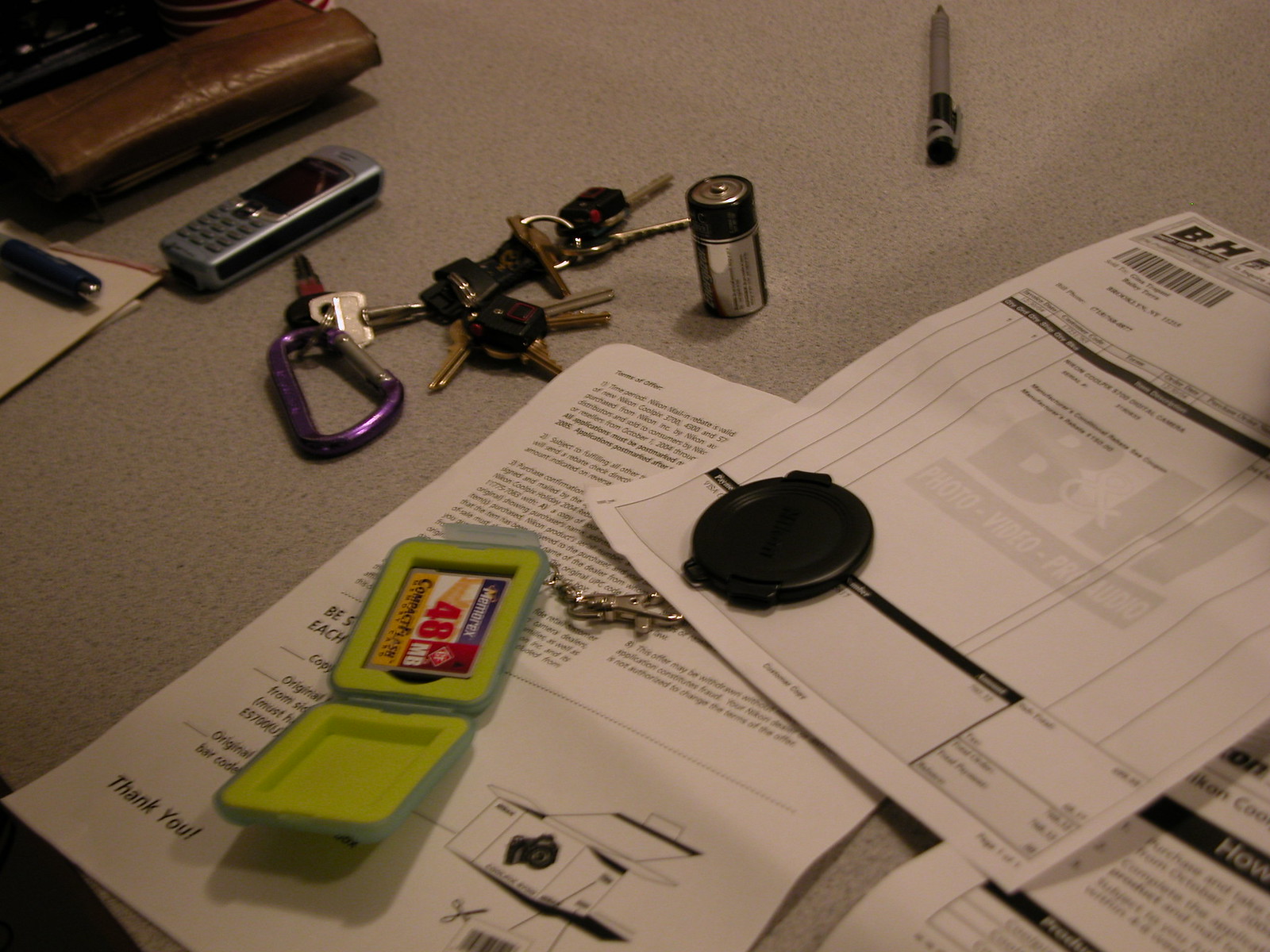On a textured tabletop, exhibiting a multi-colored sandy gray and white pattern, sits an assortment of objects arranged with varying degrees of order. 

At the top right, slightly towards the center, rests a pen with a black cap and gray body, adorned with a couple of gray stripes. The point of the pen is directed upward. 

Towards the left corner lies a leather wallet resembling a checkbook style, characterized by its longer shape. 

Descending along the left side, you will find a small notepad with blank pages, its end glued to maintain the paper's order. Resting on this notepad is a blue ballpoint pen, distinguishable by its silver clicker on the top. To the right upper corner of this pad, a compact phone, with a combination of silver and black, lies horizontally. This phone has a screen but is clearly not a smartphone. 

Moving down toward the center of the image, a set of car keys is dispersed across the table. The keyring consists of two round rings carrying approximately eight or nine keys. These keys vary in color: some are silver, others gold, with a few featuring black tops. The keys are oriented in multiple directions; a few point toward the phone while others are scattered in different directions, including one prominently pointing straight down. Attached to the set is a purple clevis hook, its orientation also downward towards the right.

Near the top right end of the key arrangement, a C or D cell battery stands on its end. The battery is silver with a black band around it and a silver top.

In the bottom right corner, several white pages of regular notebook size are visible, imprinted with black text. The visible top page is an invoice from B&H. 

In the left lower corner, there's a black lens cover partially visible, and overlapping it is a white page of instructions, ending with the text "Thank you again." On top of these instructions lies an open green hard case, which reveals a card marked with "48 MB," secured by a silver clip at the top end.